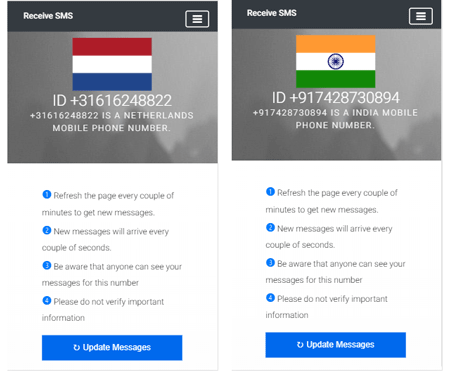Here are two side-by-side mobile device screenshots showcasing a webpage designed for receiving SMS messages. Both images lack distinguishing device interface elements, making it unclear whether they are from iOS or Android systems. 

**Left Screenshot:**
- **Page Header:** "Receive SMS" is displayed in white font on a black background.
- **Menu Button:** Located in the upper right corner, it features three horizontal lines in a rectangle with rounded corners and a white border.
- **Main Section:**
  - **Flag & Identifier:** The Netherlands flag is prominently shown.
  - **Phone Number:** Below the flag, a Netherlands mobile phone number is displayed, prefixed with "ID+".
  - **Advantages:** Various benefits are listed beneath the phone number.
- **Footer:** At the bottom, an update messages button is depicted as a circular arrow looping back to its tail, with white text on a blue background.

**Right Screenshot:**
- **Page Header:** Identical to the left, "Receive SMS" is indicated in white text on a black background.
- **Menu Button:** Matches the left screenshot with the same icon and placement.
- **Main Section:**
  - **Flag & Identifier:** Displays the Indian flag.
  - **Phone Number:** An Indian mobile phone number follows, also prefixed with "ID+".
  - **Advantages:** Lists the same benefits as the left screenshot.
- **Footer:** An update messages button like seen on the left, marked by a circular arrow icon, white text, and a blue background.

In summary, both screenshots serve as regional variants of a webpage facilitating SMS receipt, differing only in the flag and phone number displayed (Netherlands and India, respectively), while maintaining consistent design elements and functionality.